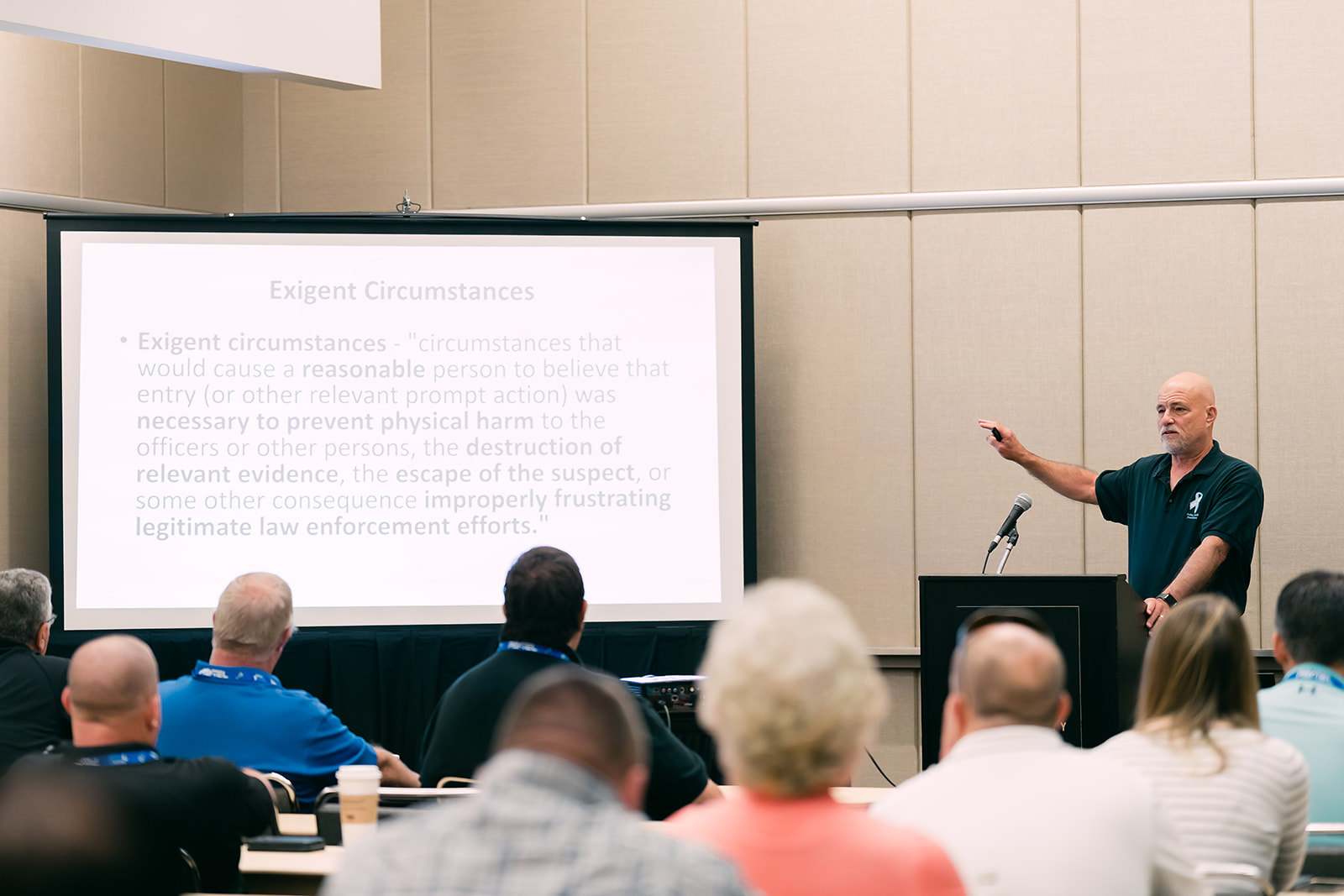In an indoor setting, a photograph captures a lecture scene where a balding, bearded man with a gray mustache, dressed in a dark blue short-sleeved shirt, stands behind a black podium equipped with a microphone. He is using his right hand to point at a screen located in the corner of the room. The screen displays text on a white background, including the phrase "exigent circumstances" and an explanation defining these as situations requiring immediate action to prevent harm, destruction of evidence, escape of a suspect, or to avoid frustrating legitimate law enforcement efforts. The audience, consisting of around ten individuals aged between 40 to 80, is seated at rows of tables, with their backs towards the camera, all attentively looking at the screen. The room features light brown paneled walls, adding to the formal setting of the presentation.